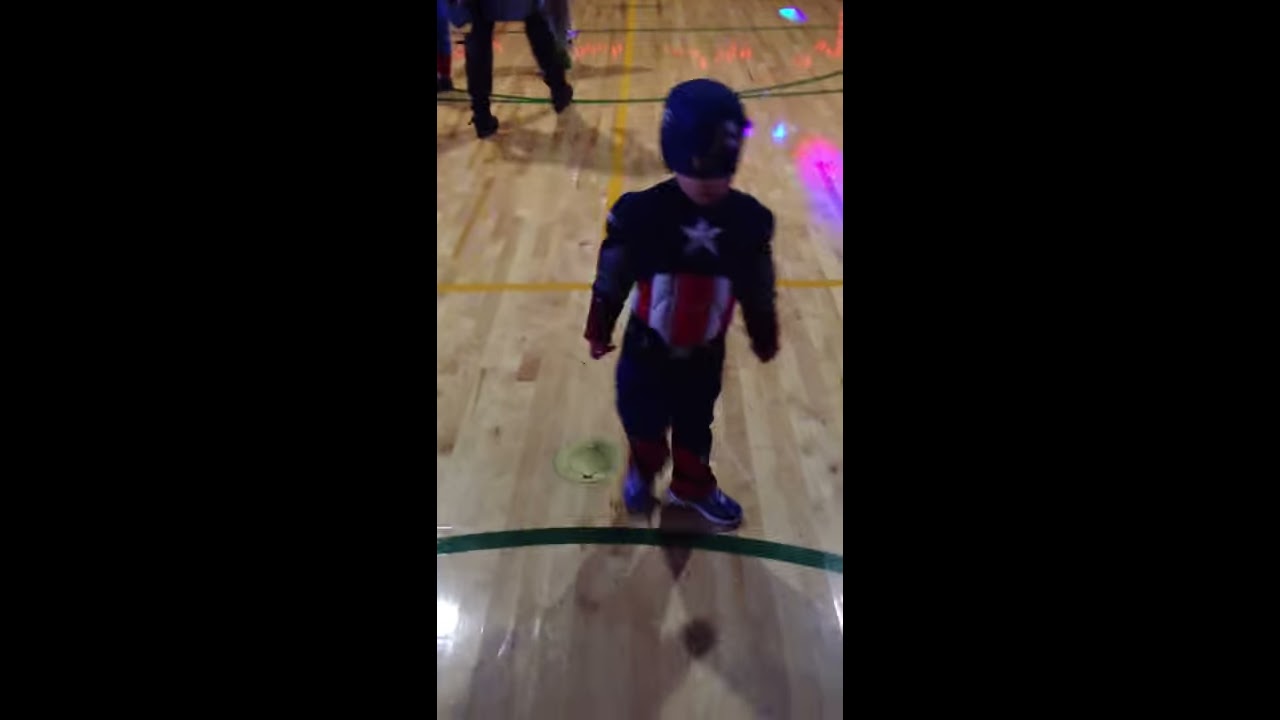The image is a color photograph in portrait orientation, set against a black landscape background. In the central section, a young boy stands on a shiny light-oak gymnasium floor, possibly a basketball court, indicated by the visible wooden planks and free-throw lines. The boy is donned in a Captain America costume, complete with a protective helmet and shield covering his face. His outfit consists of a long-sleeved top with a prominent white star on the chest and red and white vertical stripes beneath it, paired with dark trousers and blue sneakers. The photo is slightly blurred and captures reflections of pink and blue lights on the floor, hinting at a festive setting, perhaps a Halloween party. In the background, partially visible are the legs of an adult male, cropped at the waist, enhancing the image's realistic and representational photographic style.